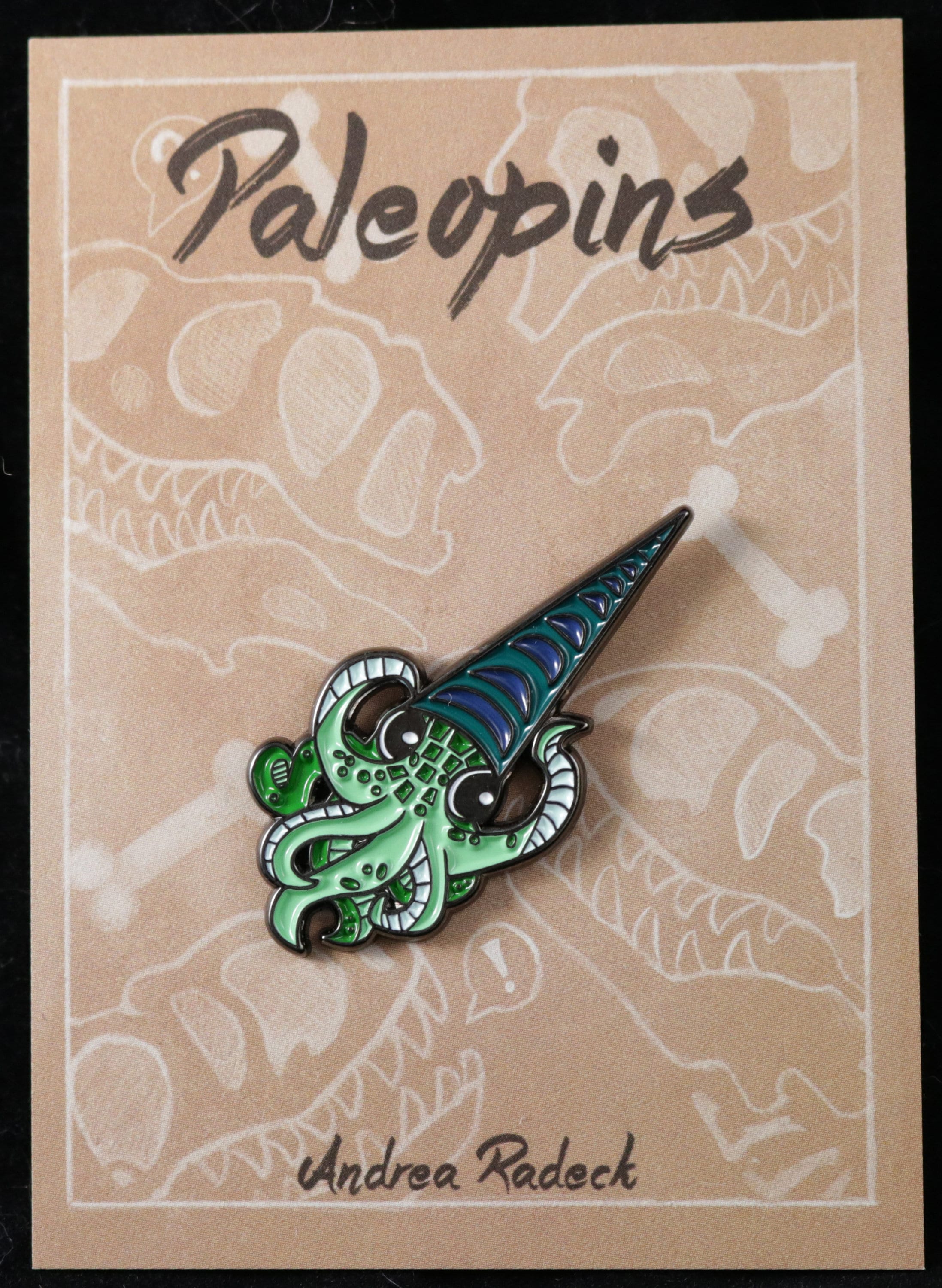This image features a beautifully detailed photograph showcasing a pin against a tan craft paper background with white illustrations of dinosaur skeletons and other prehistoric elements. Encased in a black frame, the central pin is a striking, animated depiction of an octopus. The octopus, primarily light green with darker green scales and accents, displays large, expressive black eyes accented by white. The octopus is adorned with a pointed, striped seashell hat in hues of dark blue and dark green. At the top of the image, the word "PaleoPins" is prominently displayed in a stylish dark brown font, while the artist's name, Andrea Radek, appears at the bottom in dark gray. This visually arresting piece, blending elements of paleontology and marine life, could serve as an eye-catching pin design, possibly for an Etsy shop or collectible item.